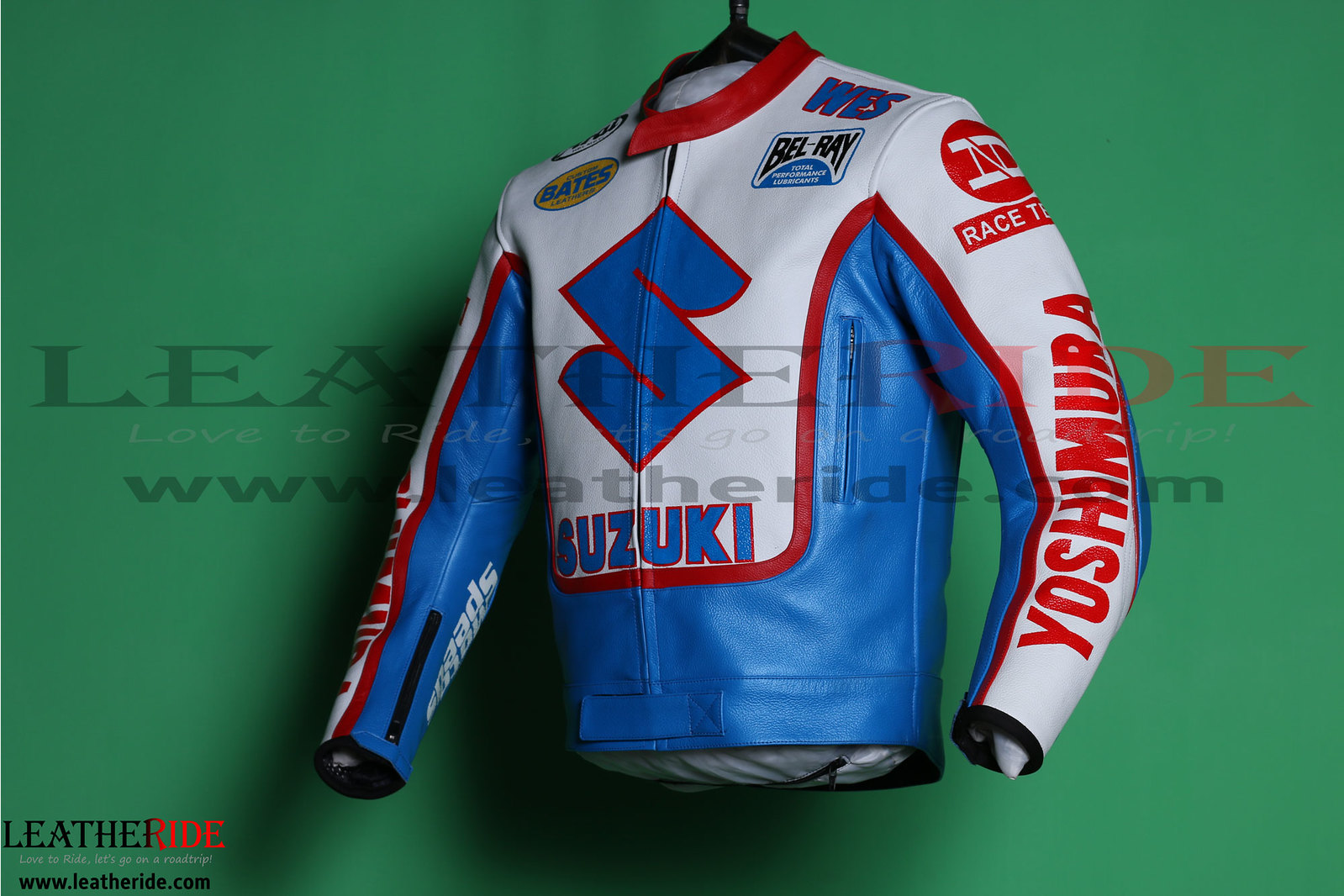A detailed photograph of a men's motorcycle jacket is set against a dark emerald green background. The jacket is prominently branded with the "Leather Ride" logo in black and red in the bottom left corner, accompanied by the URL www.leatherride.com. Both the logo and the URL reappear as a watermark diagonally across the chest area of the jacket. Positioned with the chest area facing the left side of the image, the jacket features a distinctive design: the chest and the outer portions of the sleeves are predominantly white, bordered with red. Central to the white chest panel is a large blue "S" outlined in red, with the word "Suzuki" in blue lettering beneath it. This white area continues down the outer sleeves, where the left sleeve prominently displays "Yoshimura" in red lettering. The collar of the jacket is red, while the lower section and areas underneath the arms are a deep blue, framed by red borders. The jacket appears filled out, possibly with a pillow, to showcase its shape.